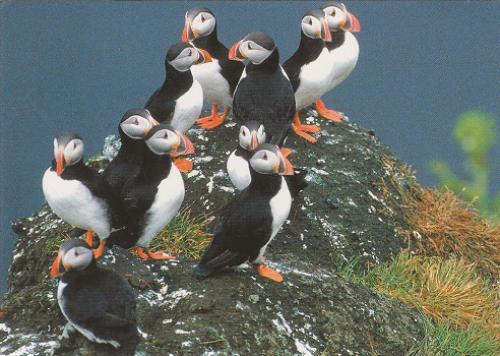The photograph features a dozen black and white penguins or possibly puffins standing atop a high, rocky hill, overlooking the sky with no visible horizon behind them. The birds, uniformly black on the back and white on the chest and belly, have distinctively bright orange beaks, feet, and legs. The rock they stand on is dark brown and heavily speckled with white, which appears to be either snow or a part of the rock itself. Patches of green and brown grass grow from the cracks in the rock, with some areas showing dead foliage, especially towards the bottom. The background of the image is a soft, blurry light blue, suggesting a clear sky or distant ocean. Notably, the penguins are arranged in groups: at the very top of the rock, five penguins are positioned with three facing right and two facing left. Just below them, another group of five has four birds looking right and one facing forward. A solitary penguin stands at the bottom left of the rock, gazing towards the left edge of the image. Their consistent size and coloring emphasize the uniform appearance of these seabirds, with white markings around their eye area complementing their stark black and white plumage.